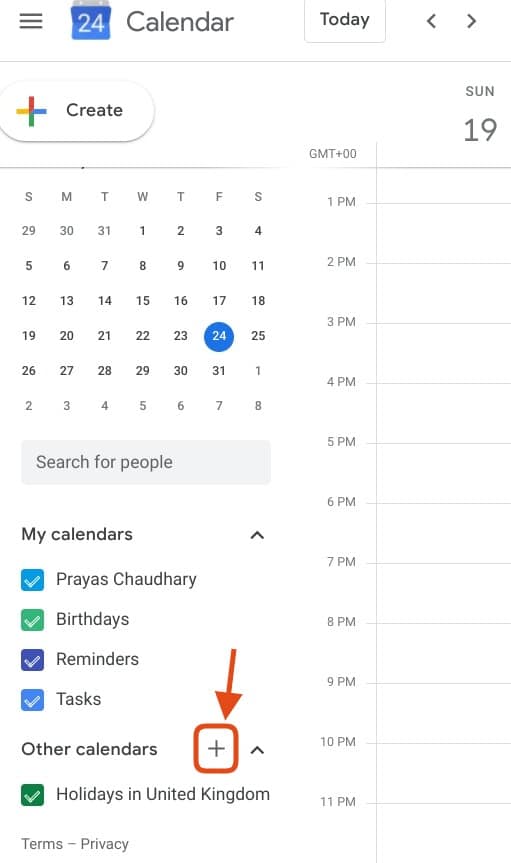The image showcases a user interface with a white background. In the top left corner, there is a hamburger menu icon next to a blue box that reads "24 Calendar." Adjacent to it are left and right arrow buttons, with a light gray bar below containing a plus symbol and the word "Create." The date displayed is Sunday, the 19th. 

Below the date, on the left side, there is a map and a note stating significant dates: the first Wednesday of the month and Friday, the 31st. The calendar view includes the days of the current month, the last week of the previous month, and the first week of the next month. 

At the top, there is a search bar labeled "Search for People," along with various calendar options such as "My Calendar," "Birthdays," "Reminders," "Tasks," and under "Other Calendars" it lists "Holidays in the United Kingdom" and "Privacy Settings."

On the right side, the calendar grid spans from 1 PM at the top to 11 PM at the bottom, structured into columns to organize daily schedules and events.